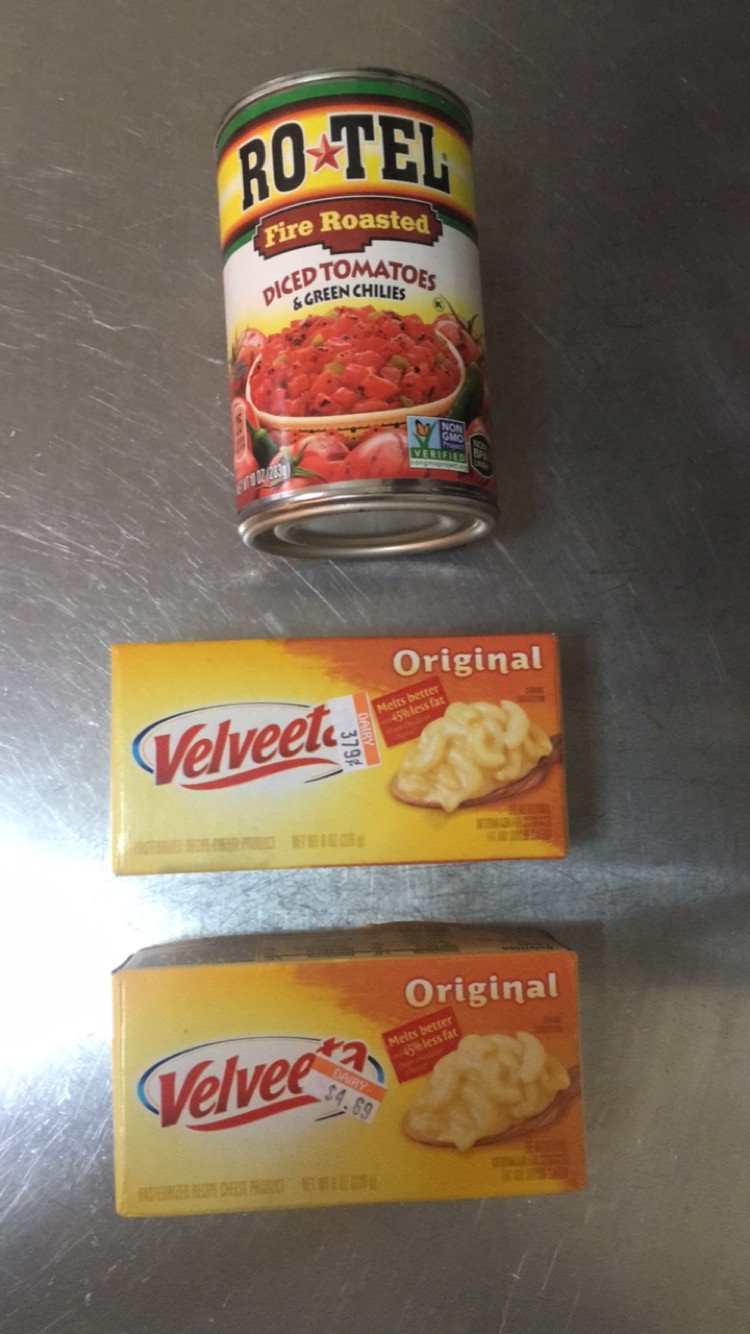The image features three distinct items placed on a gleaming silver-colored tabletop. At the top of the image is a can of Rotel, clearly labeled as "Rotel Fire Roasted Diced Tomatoes & Green Chilies." The can also indicates its size as 10 ounces. Right below the can, there's a bowl filled with the diced tomatoes and green chilies from the Rotel can. 

Below the bowl, there are two items which are blocks of Velveeta cheese, labeled as "Velveeta Original." The block on the bottom appears slightly larger than the one on top. Each Velveeta package is adorned with an image of a spoon holding creamy macaroni and cheese. The top block is priced at $3.79, while the bottom block is priced at $4.69.